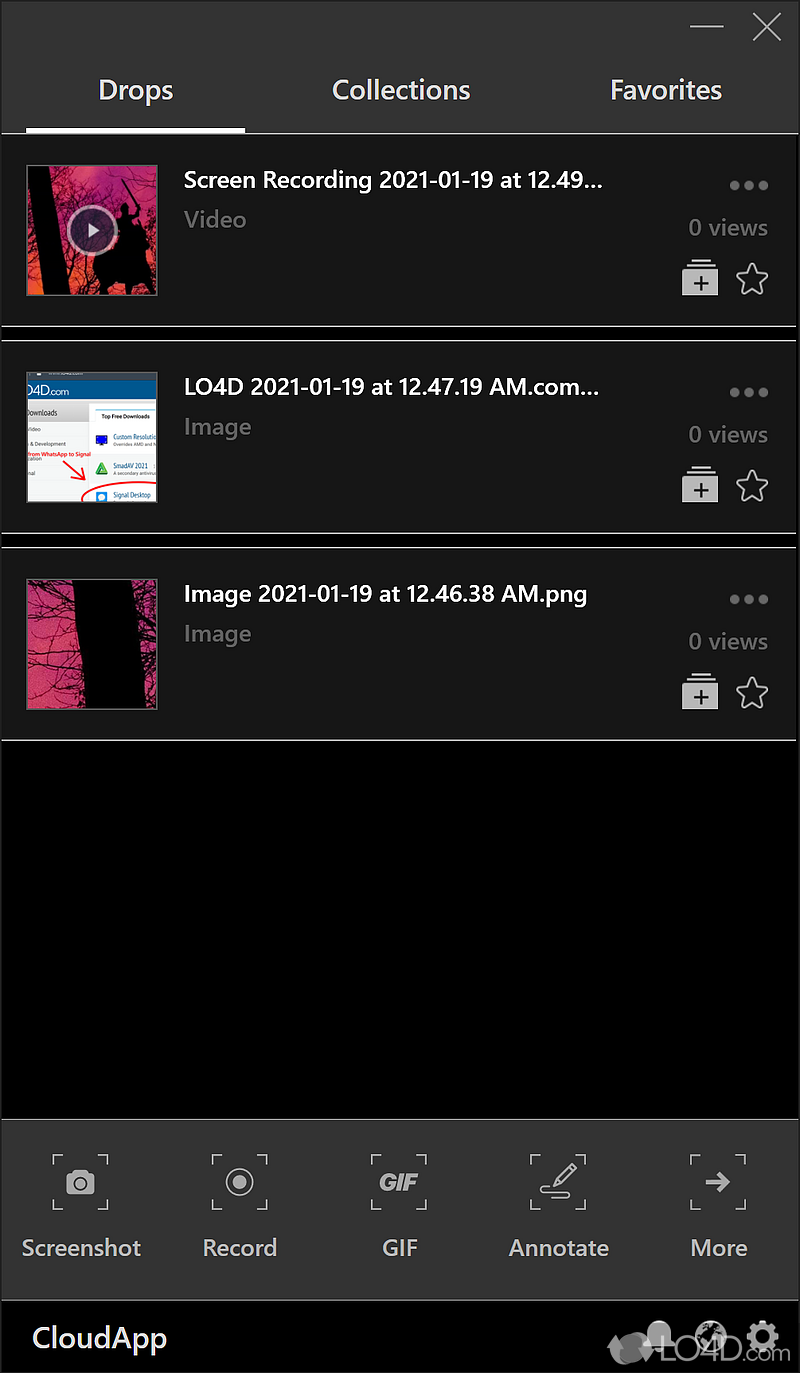This screenshot captures the interface of a dark-themed application named CloudApp. The interface features three prominent tabs at the top: "Drops," "Collections," and "Favorites," with the "Drops" tab currently active. The main content area displays a list of items under the "Drops" tab.

The first item in the list is a video titled "Screen Recording 2021-01-19 at 12.49..." which is followed by two image files—"LO4D 2021-01-19 at 12.47.19am" and "image 2021-01-19 at 12.46.38am.png." Each item is accompanied by a thumbnail image, the file type icon, and the number of views it has garnered. 

Directly below the list of items, a toolbar provides quick access to various functionalities including "Screenshot," "Record," "GIF," "Annotate," among other options. The interface is branded with a watermark from LODE.com, suggesting that the content might have been prepared or shared through this platform. 

Overall, this screenshot appears to depict a user demonstrating or sharing the CloudApp interface, possibly after uploading the image to LODE.com for further dissemination. The layout highlights the seamless and organized display of diverse media files, catering to streamlined digital asset management.